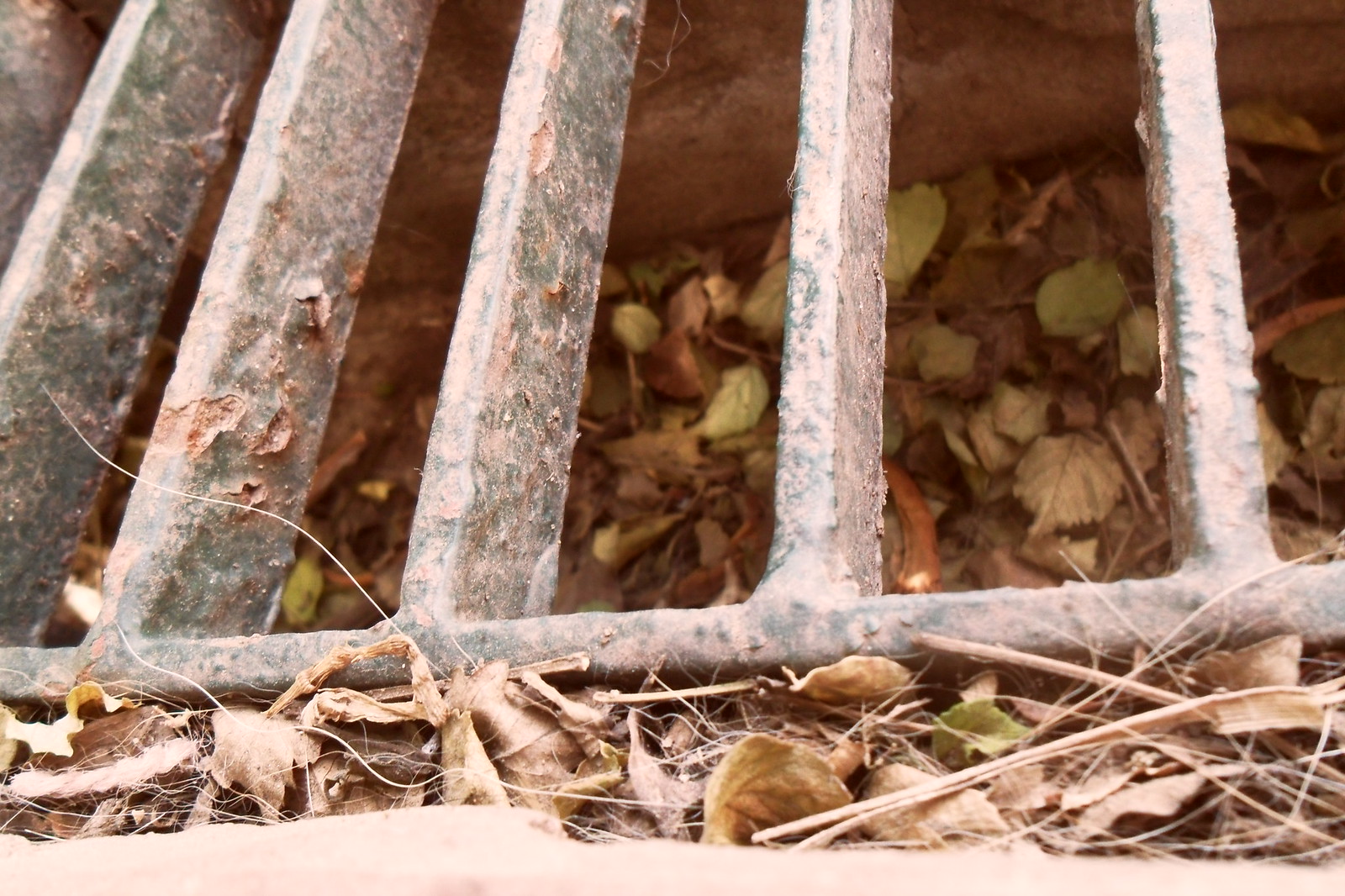The photograph captures a weathered wrought iron fence or grate, originally black but now heavily rusted, displaying various pockmarks and visible sections where the paint has flaked off, exposing brown rust and bumps. The grate is positioned horizontally, with the top half resting on a rock and the bottom half nestled in dead grass and leaves. Five rungs, welded securely to the bottom of the grate, are discernible. Among the majority of dead leaves scattered beneath and above the grate, a few retain shades of green, while some exhibit unusual blue hues and others are tinged brown and yellow. The scene suggests an outdoor setting, likely in the fall, although the exact environment remains indeterminate due to the close-up nature of the shot. Despite the ambiguity of perspective, either looking up or down, the grate is clearly old and deteriorated, adorned with cobwebs and debris.